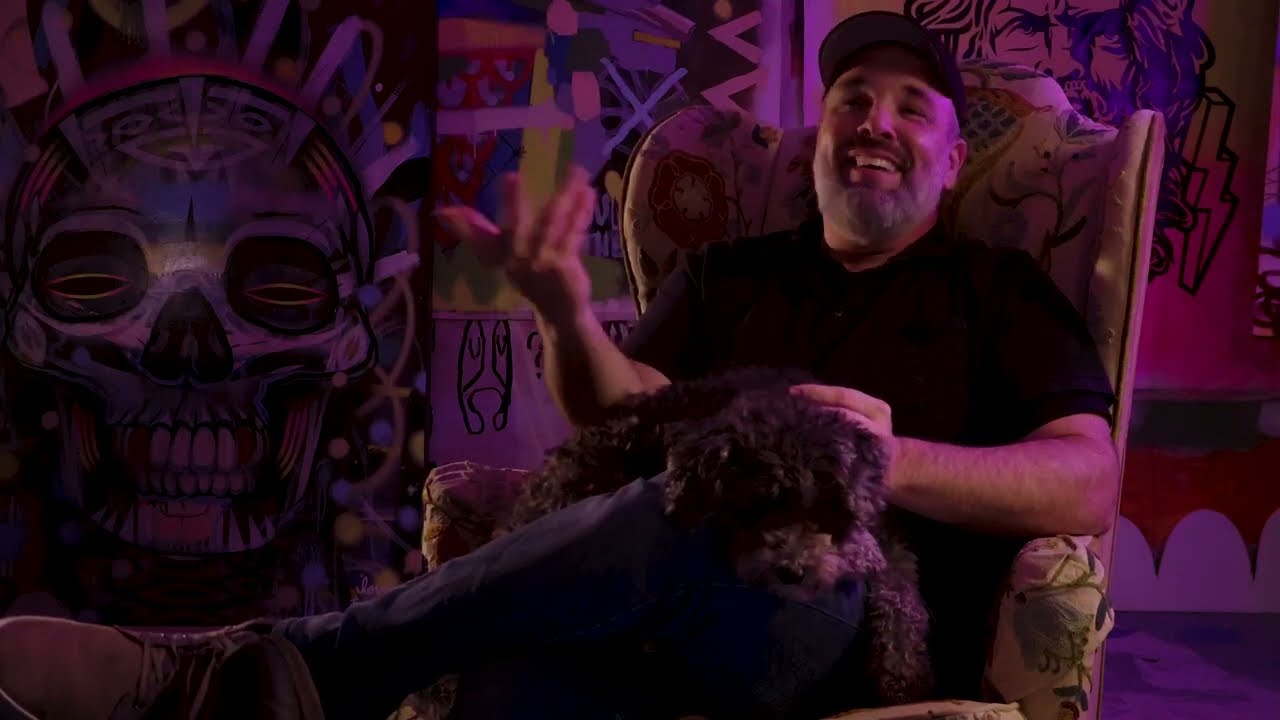The photograph captures a man seated in a high-backed chair adorned with a flower design. The ambient lighting casts a red glow over the scene, giving it a dim, somewhat dark atmosphere. The man, who has a light complexion, is wearing a black ball cap, a black t-shirt, blue jeans, and brown lace-up shoes. He's smiling broadly, looking towards the left side of the frame, with his mouth open, revealing his top row of teeth. He appears to be engaging in a conversation, with his right hand lifted and palm facing upwards while his left hand rests on a dark furry dog, resembling a poodle, on his lap.

The backdrop of the image features an eclectic mix of artistic elements. Prominently, there's a large skull with its eyes open wide and teeth showing, possibly influenced by Mexican art styles. Surrounding the skull are various graffiti-like paintings, including a comic-book-style man and a face with long hair alongside a lightning bolt. The overall setting suggests an art studio or a creative space, rich with vibrant and funky designs. The man exudes an aura of joy and contentment, making the space feel lively and inviting. His pleasant demeanor, combined with the colorful, artistic background, creates a powerful and engaging visual composition.